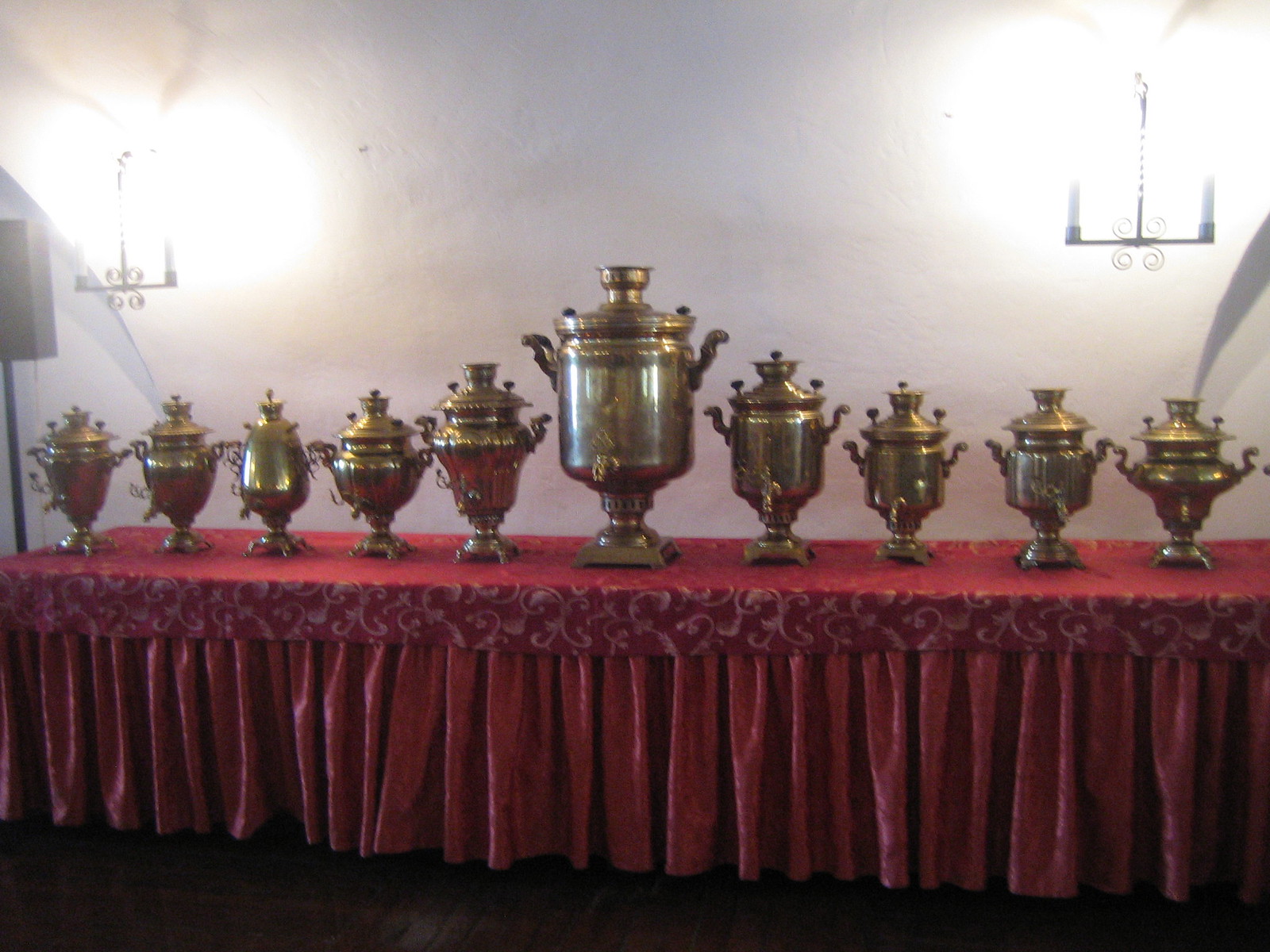The photograph captures an intricately detailed display on a long table dressed in rich red velvet, with the tablecloth pleated along the lower edge and brocaded on the upper surface. Centered on the table is a series of ten ornate brass urns, lined up in descending order of size from a very large central urn to smaller ones towards the edges. These urns, resembling traditional Indian brass containers, appear to serve as liquid dispensers, each adorned with elaborate handles that curve upwards and similarly styled lids. One urn, third from the left, stands out with its egg-shaped design amidst the predominantly rectangular or square shapes of the others. The arrangement also includes two bright lamps on the white textured wall behind the table, one on each side, casting a striking glow over the scene. The dark floor further accentuates the vibrant red tablecloth and the lustrous brass of the urns, creating a captivating and ornate tableau.